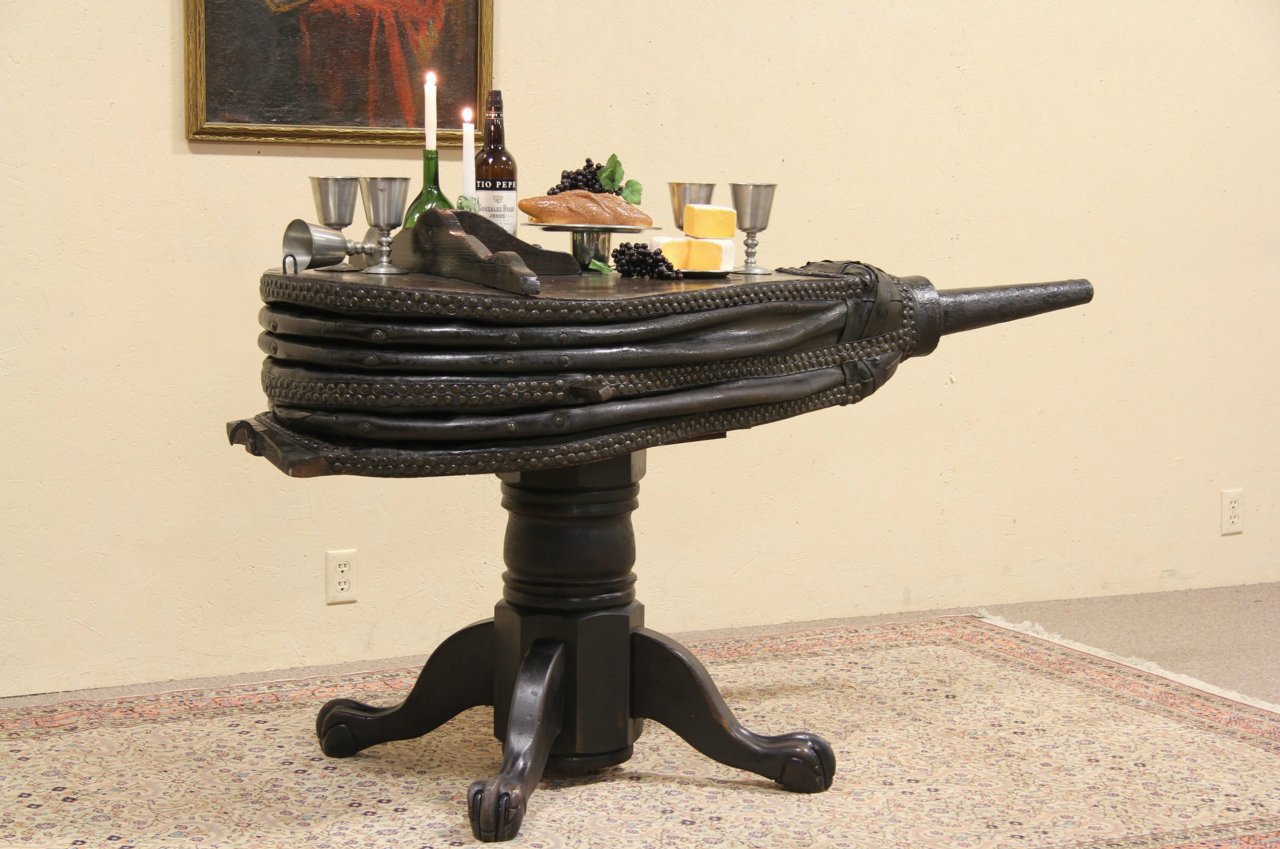The image showcases a uniquely designed, small wooden table with a dark brown, intricately carved tabletop resembling an ancient bellows, the device used to blow air onto a fire. The table stands on a sturdy central pillar with four legs resembling clawed feet. The surface of the table is adorned with an array of items: five silver goblets, with four standing upright and one laying on its side, a collection of lit candles including one in a green bottle, a bottle of wine, and an assortment of bread, fruit, and cheeses. The table is positioned on a light tan carpet with light pink borders and brown specks, set against a white wall. In the background, there's a partial view of a painting framed in gold, featuring dark brown and burnt red tones.